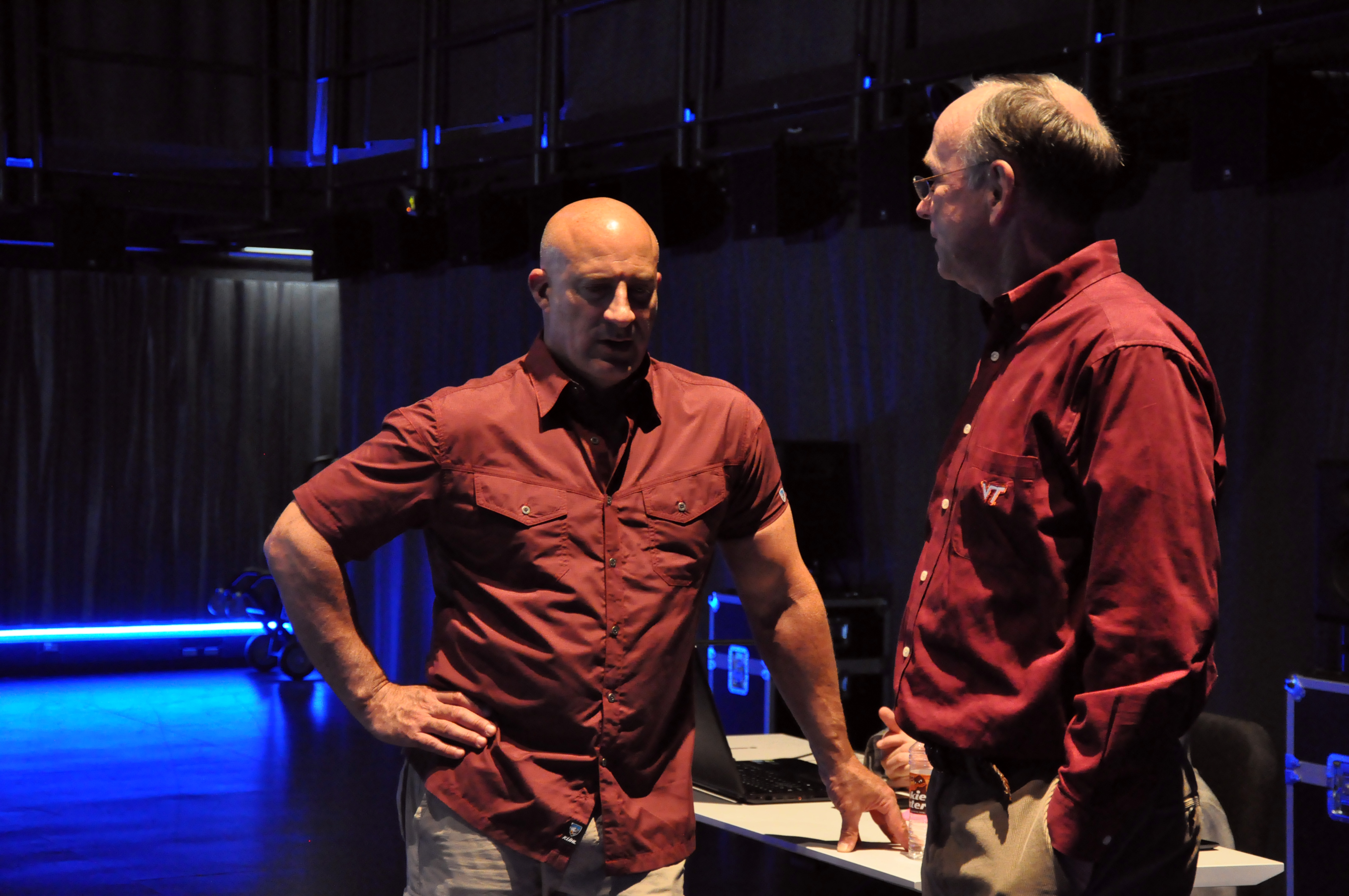In a dimly lit indoor setting that resembles a performance stage, two men are engaged in a conversation. The background is dark, but blue lights illuminate the ceiling and floor, highlighting the stage area. The man on the left, who appears to be in his 50s, stands facing the viewer. He is bald, with a short-sleeved collared maroon shirt that features pockets on both sides of his chest, and khaki pants. One of his hands rests on a white table, while the other is placed on his hip as he looks downward. The man on the right, likely in his 60s or 70s, has graying hair and is slightly balding. He wears glasses and a long-sleeved maroon shirt with "VT" on the pocket, indicating Virginia Tech. He is also dressed in khaki pants and stands facing the other man, as if they are deep in conversation.